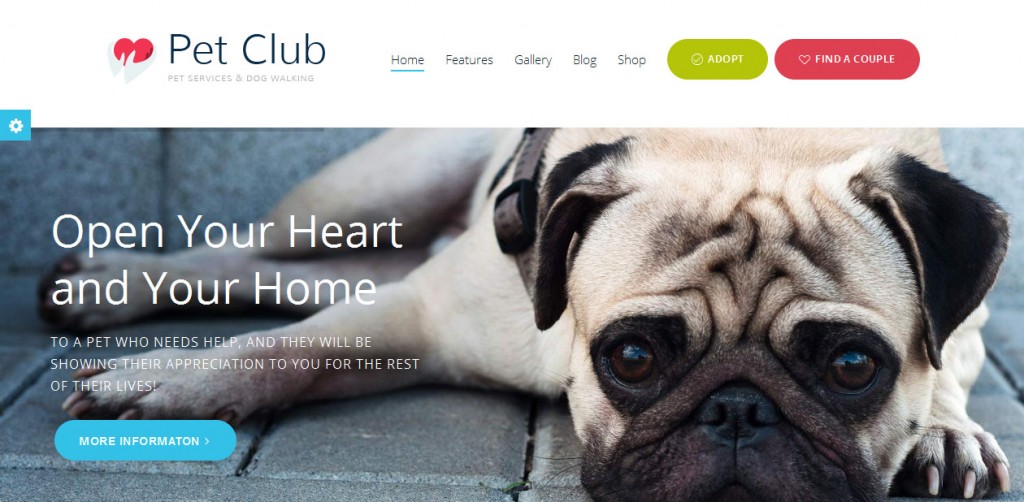A screenshot of a website page titled "Pet Club: Pet Services and Dog Walking." The website has a charming heart icon next to its title. Along the top navigation bar, there are various menu options: Home, Features, Gallery, Blog, Shop, Adopt (highlighted with a green button), and Find a Couple (marked with a red button and a heart icon).

The main image on the page features an adorable small dog, possibly a pug or French bulldog, with a wrinkled snout and forehead. The dog, which is brown in color, is lying on a sidewalk and appears to be wearing a body harness. To the left of this cute pooch, a heartwarming message is displayed: "Open your heart and your home to a pet who needs help. They will show their appreciation to you for the rest of their lives."

Below this touching message is a blue button labeled "More Information," inviting users to click for further details. In the top left corner of the image, there's a small settings icon represented by a gear, presumably to adjust website preferences. The overall layout and imagery create a welcoming and loving feel, reflecting the theme of Pet Club.